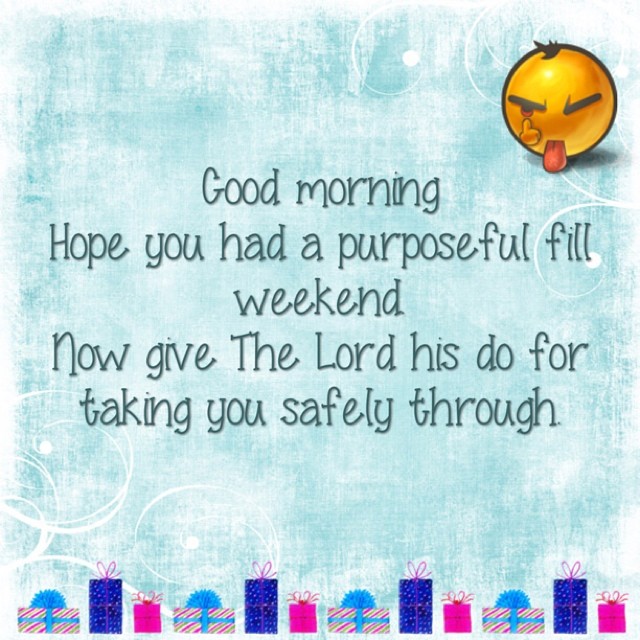The image is a 5-inch by 5-inch computer-generated meme with a light teal and white, slightly faded background featuring white curves and swirls. At the top, there is a cheerful yellow emoji in the upper right corner, giving a thumbs-up with one eye open, its tongue sticking out, brown spiky hair, and raised eyebrows. The main text reads, "Good morning, hope you had a purposeful Phil weekend. Now give the Lord his due for taking you safely through," written in a dark green, comic-style font. The lower portion of the image showcases a repeating pattern of cartoon gift boxes forming a border: one in diagonal striped paper with a blue ribbon, a tall narrow dark blue box with a pink ribbon, and a smaller square pink box with a red ribbon.